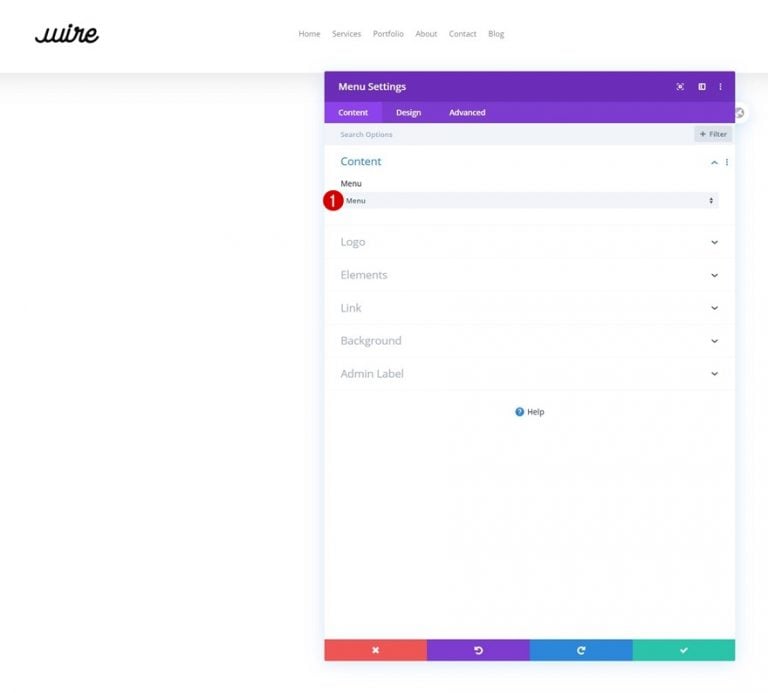This is a screenshot from the website "WIRE," which offers services of an unspecified nature. The website's name "WIRE" is displayed in an ornate, cursive font where all the letters are interconnected. At the top of the page, there are six navigation titles in a small, grey font: Home, Services, Portfolio, About, Contact, and Blog. 

The user has accessed the menu settings, which appear over a purple background with white text. The opened menu reveals the content tab, indicating one red notification beside the "Menu" option. Additional notifications can be seen next to the options labeled "Logo," "Elements," "Link," "Background," and "Admin Label." A help section is also visible, marked by a blue question mark that users can click for further support.